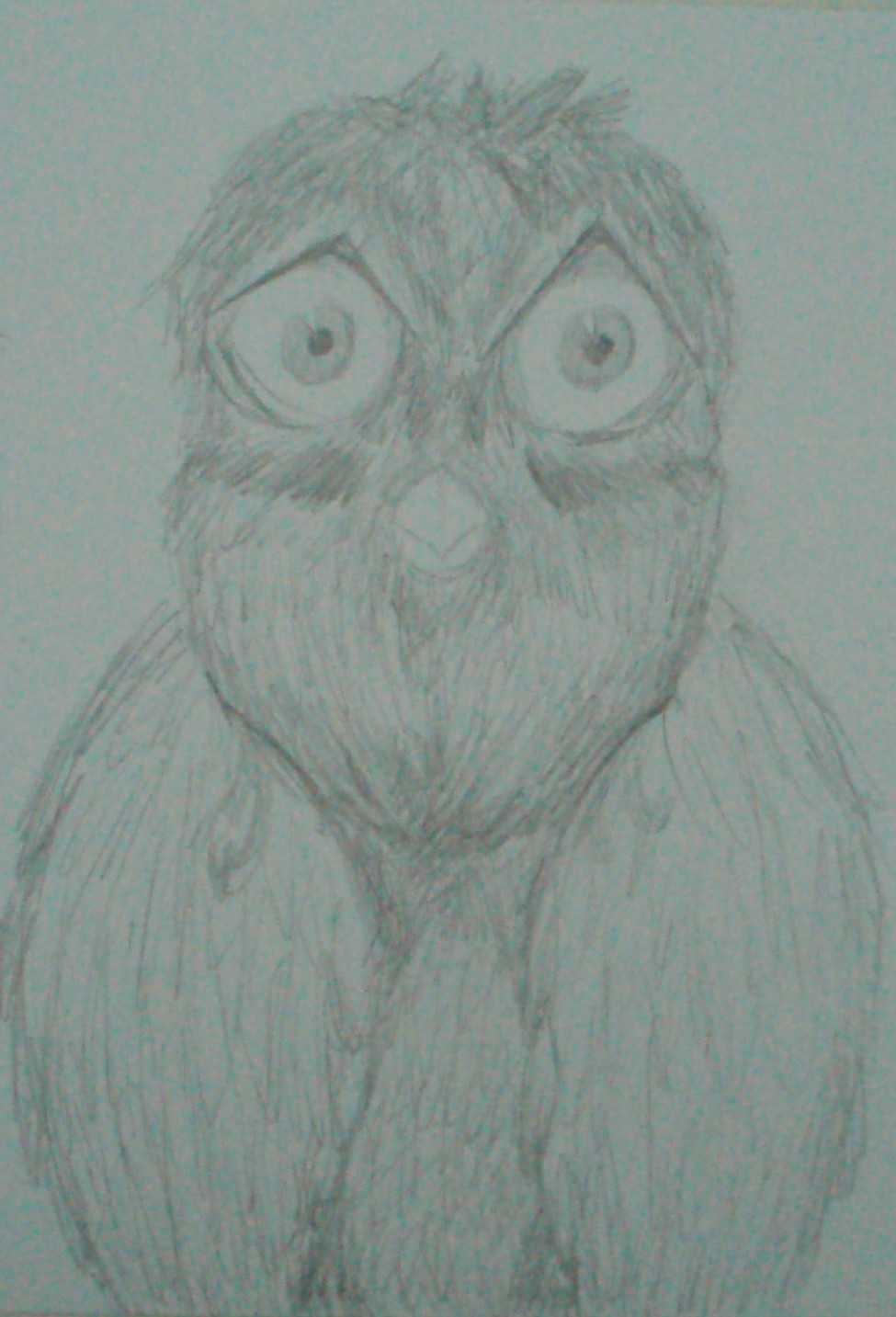This is a pencil drawing on a grayish, bluish, greenish, and somewhat splotchy background, depicting what appears to be the face of an owl. The drawing features a highly detailed feathery head with feathers or hair sticking up at the top. The owl's sizable, expressive eyes dominate the composition, characterized by large whites, big irises, and large pupils, with the tops of the eyes forming pointed triangles and shadows underneath them. The beak is evident, though not colored in, situated between the striking eyes. The artist has shaded under the chin and sketched detailed feathers around the eyes and on the breast area. The owl's wings are visible extending to either side, suggesting the shoulders and partially down the body, accentuating the feathered texture.